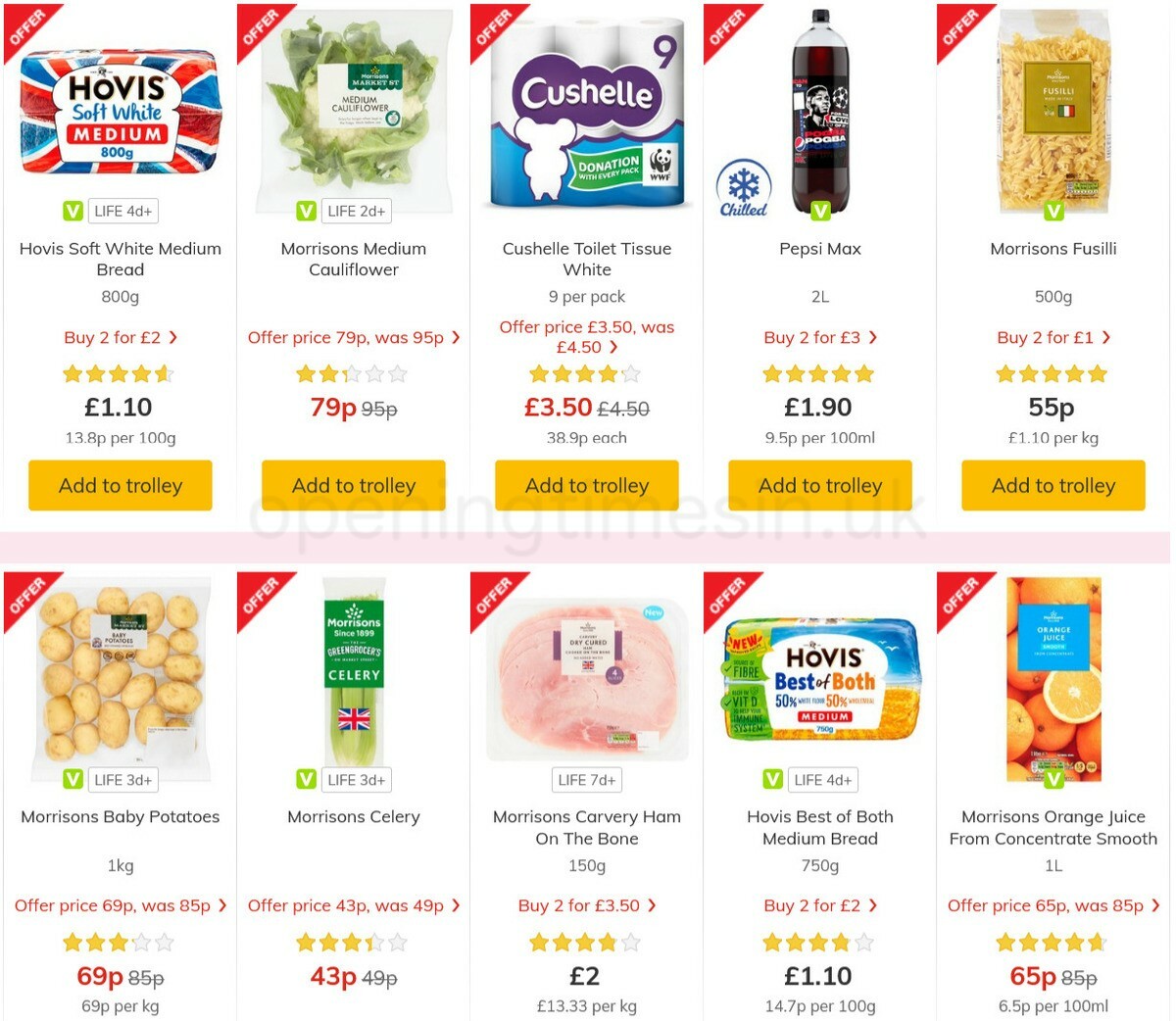A screenshot of various sale items from an unidentified grocery store is featured in this image. The currency used is pounds (£). The items and their promotional prices are displayed in a virtual shopping app, possibly similar to Instacart. The sale items include:

- Hovis Soft White Medium Bread, available for £2 when you buy two loaves.
- Morrison's Medium Cauliflower, now priced at 79p, down from 95p.
- Cushel White Toilet Tissue, priced at £3.50.
- Pepsi Max, offered at £1.90.
- Morrison's Fusilli, available for 55p.
- Morrison's Baby Potatoes, priced at 69p.
- Morrison's Celery, costing 43p.
- Morrison's Carvery Ham on the Bone, priced at £2.
- Hovis Best of Both Medium Bread, also on sale.
- Morrison's Orange Juice from Concentrate (Smooth).

The app interface suggests users can easily add these items to their trolley or basket, emphasizing the convenience and variety of sale options available.